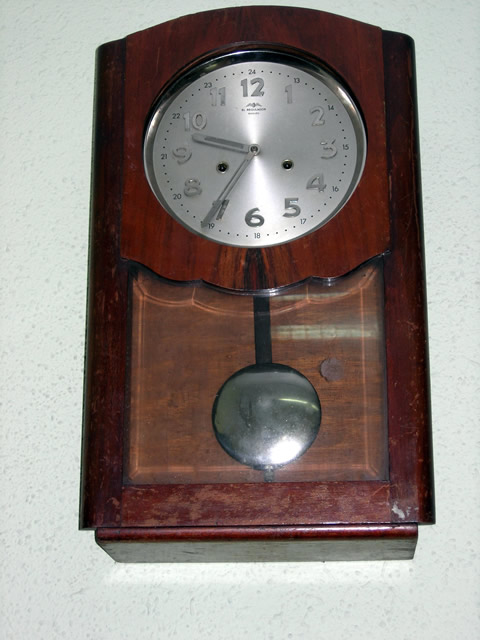Displayed against a light gray wall, this image features an antique wooden clock with a dark brown, polished finish that exudes a shiny, nearly oily appearance. The clock's structure is a long, rectangular form with an elaborately curved top. In the center of the clock, there is a circular glass-covered opening, revealing the silver clock face adorned with silver numbers from 12 to 11. The clock hands—both silver—show the long hand pointing to the 7 and the short hand resting between the 9 and 10. Below the clock face, a large silver pendulum with a rounded bottom and vertical stick attachment is visible through another glass section. The clock's rich wooden frame, coupled with its intricate details and classic design, suggests an old-fashioned, possibly antique piece.